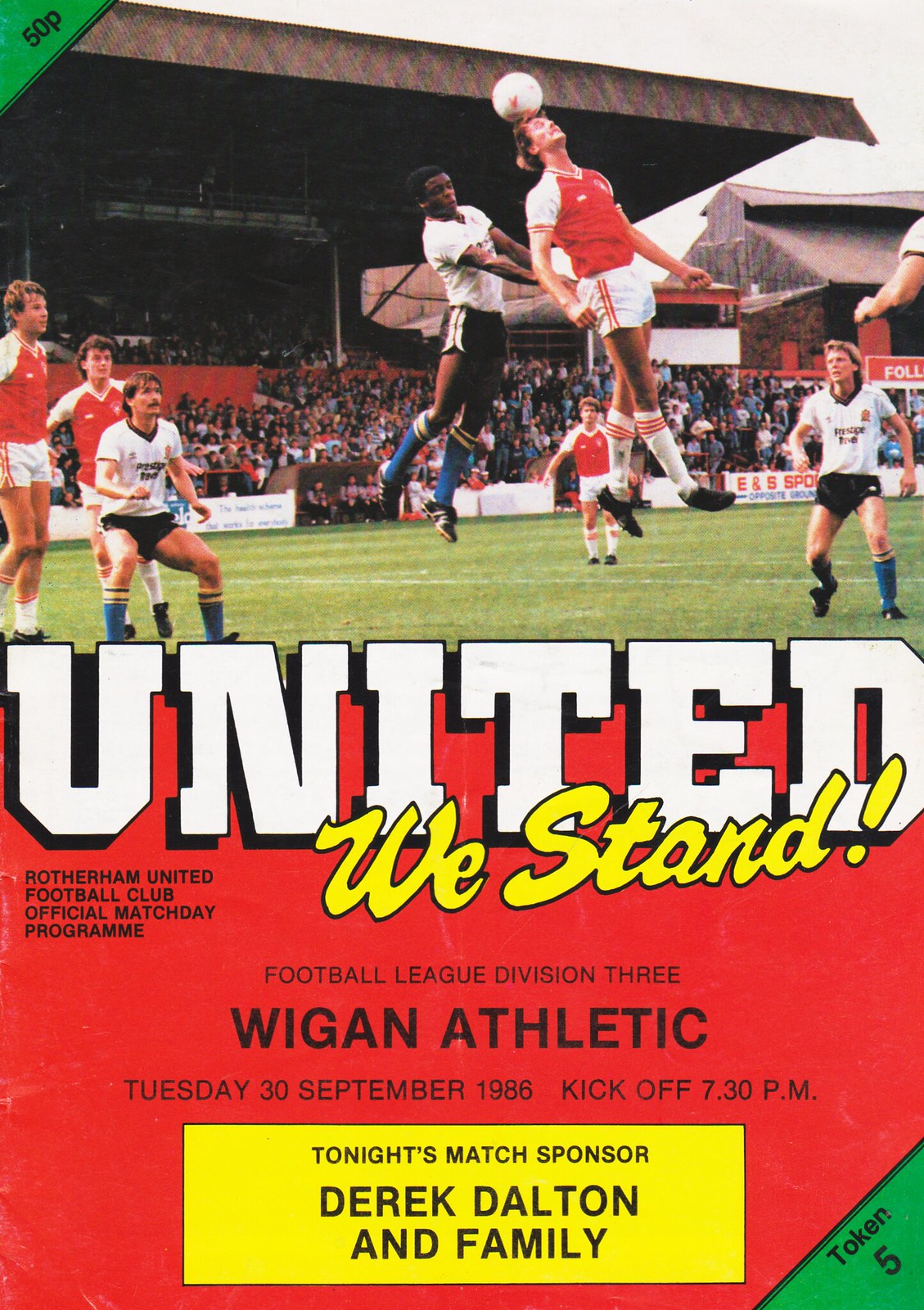This magazine cover serves as an official program for a football game, prominently advertising a Football League Division III match featuring Wigan Athletic, scheduled for Tuesday, 30th September 1986, with a kickoff at 7:30 pm. The cover's top half showcases a vivid action photograph set on a grass field, capturing the intense moment when a player in red and white is leaping about three feet in the air to head the soccer ball, while an opposing player in white and black, with outstretched arms, closely contests the play from behind. Other players are scattered around the field, with spectators filling the stadium's stands in the background. The top left corner of the cover features a small triangle marked with "50P", indicating the price. Above the photograph, stadium signage reads "ES Sports", adding to the authentic game day atmosphere. The central portion of the cover boldly states, "United We Stand!" in large white lettering against a red background, symbolizing unity and team spirit. Beneath this, crucial match details are provided, and a yellow box at the bottom highlights, "Tonight's Match Sponsor, Derek Dalton and Family", celebrating the sponsorship support.